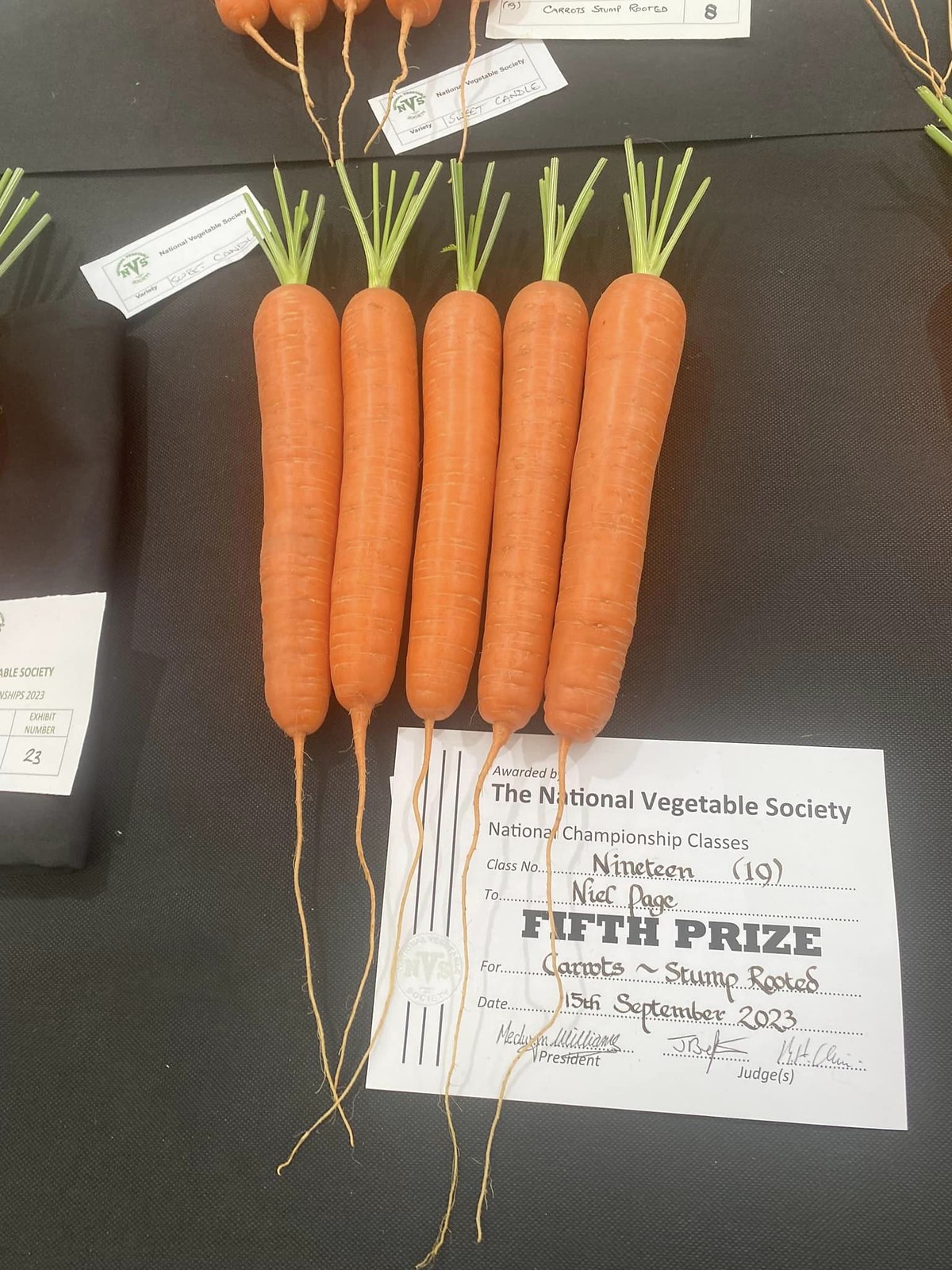The photograph depicts a food growth contest setting, likely at an indoor event such as a state fair or farmer's market. Central in the image are five carrots laid out in a row on a table with a dark black background. Each carrot displays vibrant green leafy tops and elongated, stringy roots that dangle over the table's edge. Below the carrots is a prominently visible white placard indicating that the judging is organized by the National Vegetable Society. The placard reads: "National Championship Classes, Class Number 19, Awarded to Neil Page for Carrots Stump Rooted, 5th Prize, Dated 15th September 2023," and includes signatures from both the president and judges. The detailed display highlights the significance of the event and the specific achievement in vegetable cultivation, with references to other prize-winning displays in proximity.